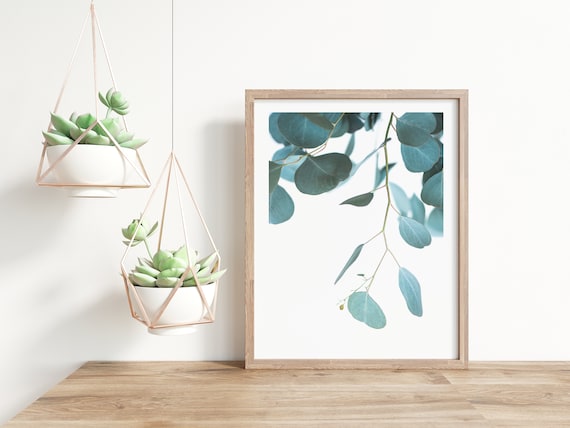The photograph features a light wooden table against an off-white wall. Leaning slightly against the wall on top of the table is a framed painting of simple greenish leaves with a white background. The wooden frame of the painting matches the table's light wood tone. To the left of the painting, two hanging succulent plants in white bowls are suspended from the ceiling by decorative geometric wooden holders. These holders consist of thin wooden pieces arranged in triangular shapes. The succulents are a soft light green, adding a touch of natural elegance to the minimalist setting.